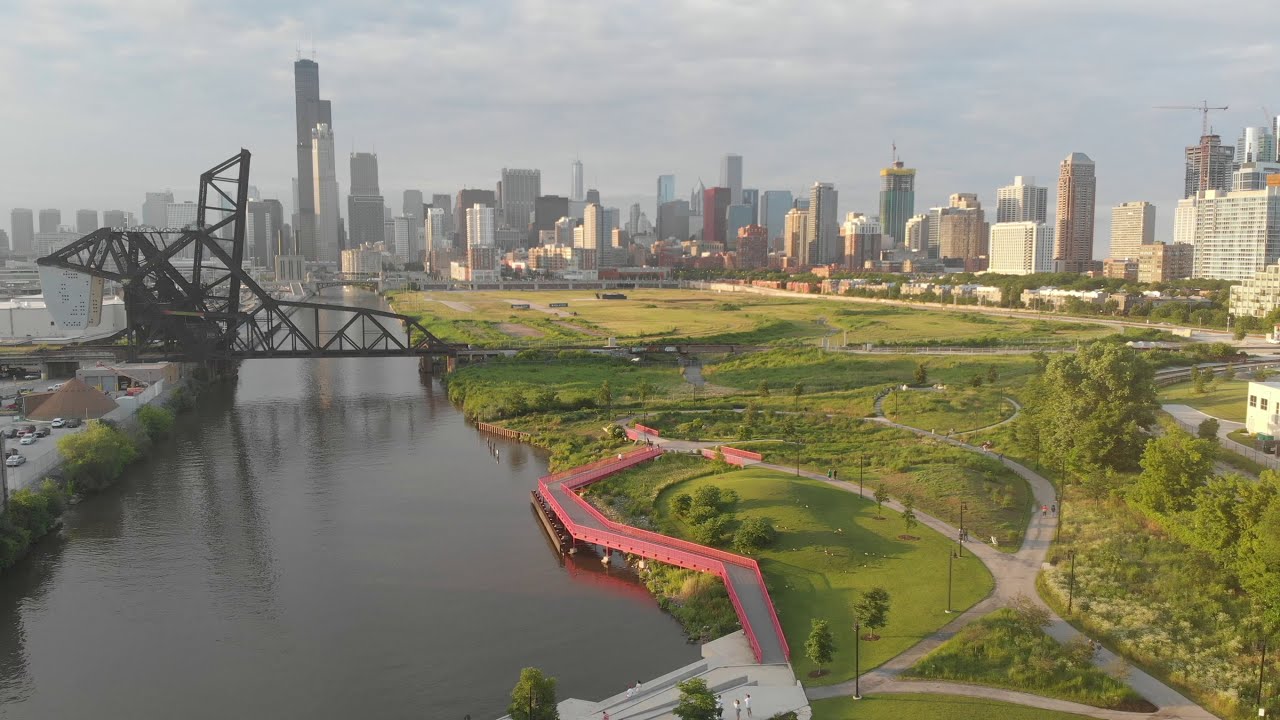This aerial drone capture showcases a vibrant cityscape featuring a harmonious blend of urban and natural elements. Dominating the scene is an expansive, verdant park characterized by abundant trees, lush grass, and intersecting pathways for pedestrians. In the park’s vicinity flows a serene river, spanned by a prominent black drawbridge, facilitating easy crossing. A unique red bridge is also visible, likely intended for smaller vehicles or pedestrian use. 

To the left of the park, the river's meandering course is clearly visible. The park creates a striking contrast to the adjacent urban area, marked by a bustling industrial zone. On the opposite side, an impressive array of skyscrapers, including some under construction with visible cranes, defines the city skyline. The iconic silhouette of what could be the John Hancock building hints at the possibility that the city is Chicago. 

Additional points of interest include a small structure reminiscent of a garage near a parking lot area, and a triangular building-like formation, possibly under development or used for storage. The scene is bathed in diffused daylight, with partial sunlight filtering through patches of gray, hazy clouds casting a calm, subdued light over the cityscape. People can be seen at ground level, contributing to the lively yet tranquil atmosphere of the urban park.